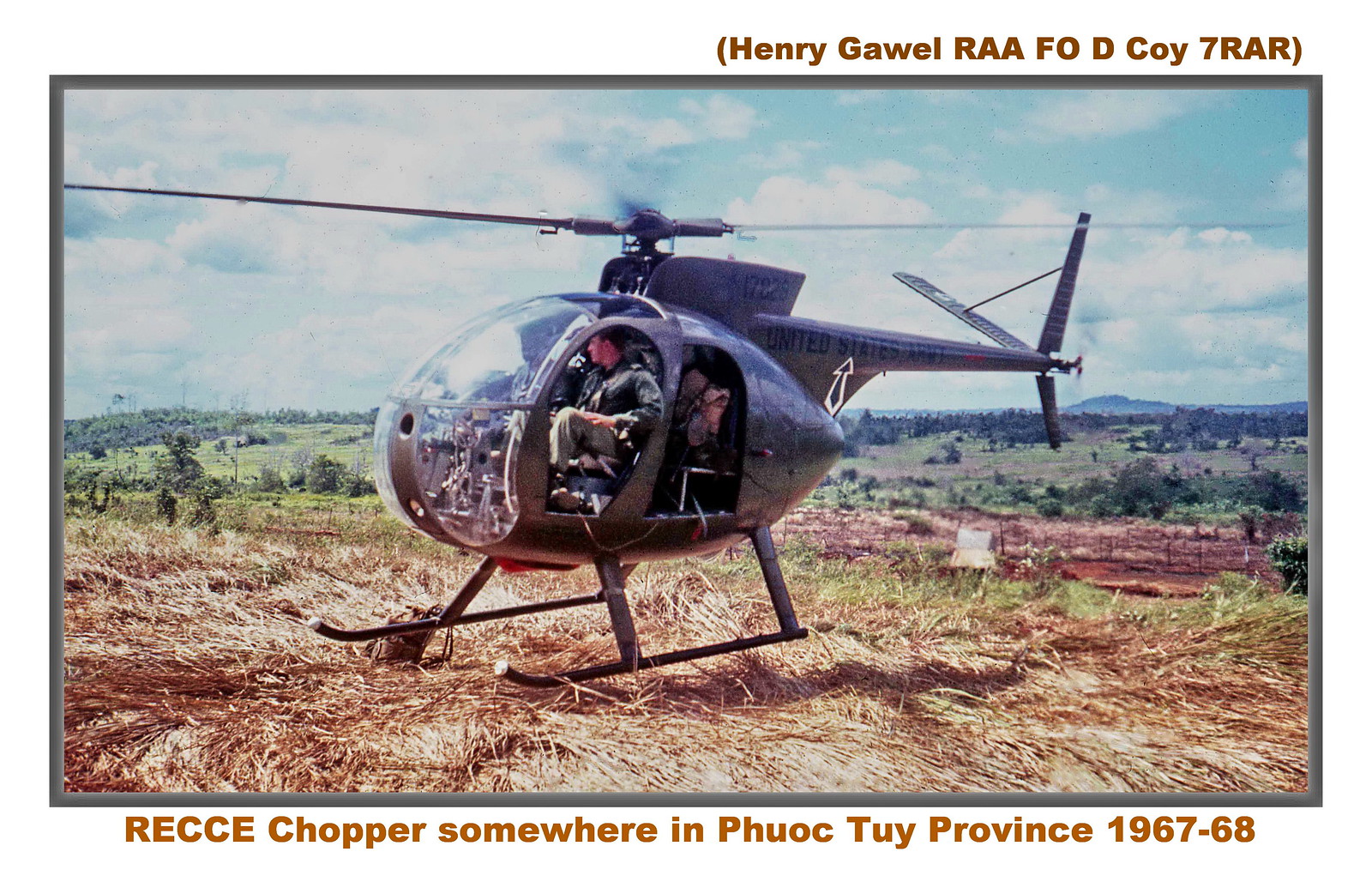The image depicts an old military helicopter from the Vietnam War era, seemingly either landing or taking off in a grassy field. Marked "United States Army" on the tail, the helicopter is the centerpiece of the photograph. Inside the chopper, at least two individuals in military uniforms can be seen at the controls. The helicopter hovers just above the brown grass under an overcast sky, with white clouds and a blue sky stretching across the top half of the scene. The landscape in the background features small trees, possibly a low-rise hill, and appears to be agricultural land.

The photo is framed by a solid white border, with text captioning both above and below the image. The top text, in brown color, reads "Henry Gowell, R-A-A-F-O-D, C-O-Y-7 R-A-R." Below the picture, a lighter brown caption says "RECCE chopper somewhere in Phuoc Tuy Province, 1967-68," indicating the location and time period. The overall setting appears to be the outdoors, likely in Vietnam, during the period of 1967-1968 in Phuoc Tuy Province.